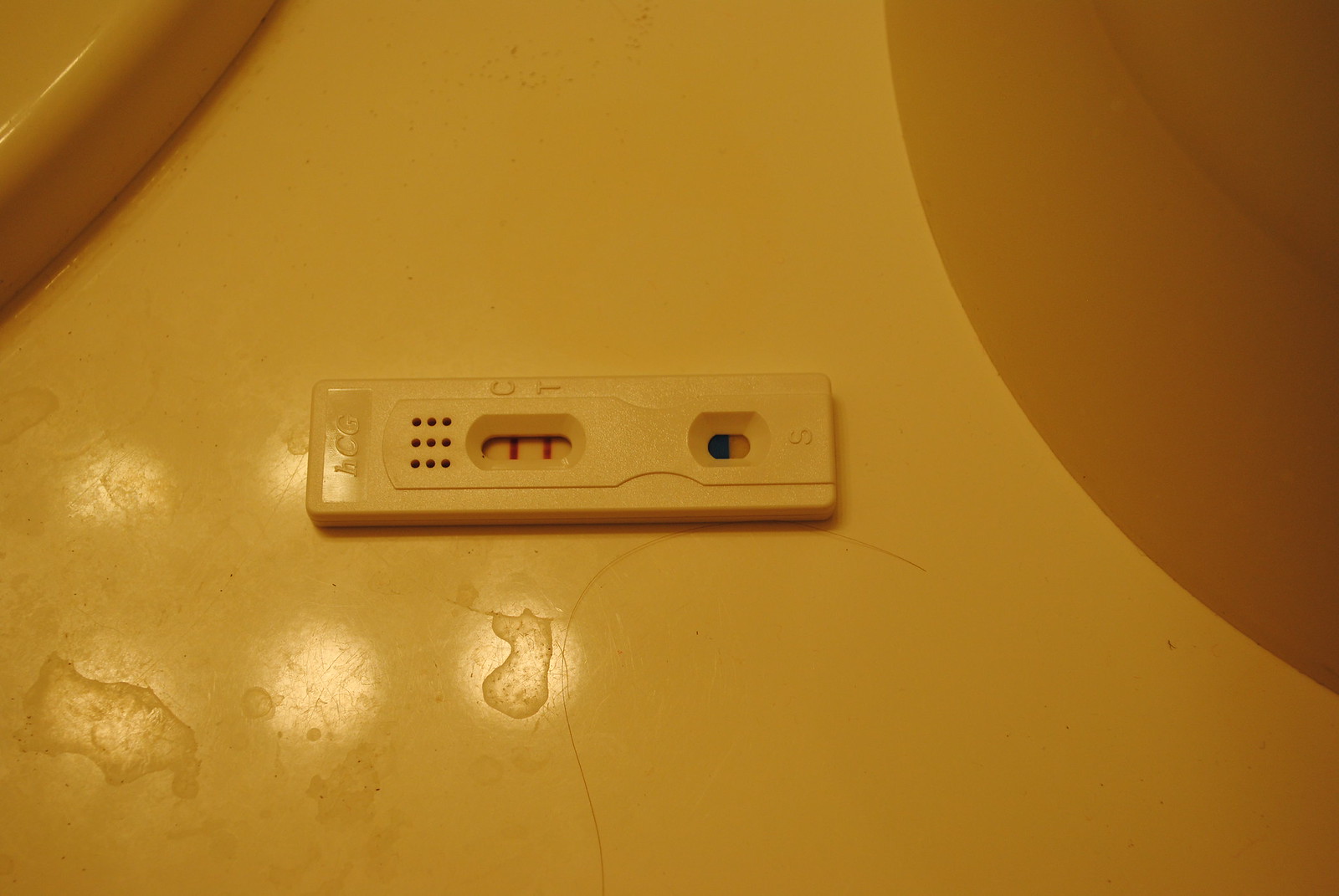The image features a small, white, rectangular testing device, possibly a pregnancy test. The central part of the device displays two parallel red lines; the left line is labeled 'C' and the right line is labeled 'T.' To the left of these red lines are approximately nine black dots arranged vertically. To the right of the red lines, there's a partially green indicator on the left side, transitioning to white on the right. Additional markings are visible; on the far left side, there are letters that appear to read 'HCG' or possibly 'HC6.' On the bottom right side of the device, there's a sideways letter 'S.' The device is situated on a white countertop. Partially visible in the background are a purple-colored plate in the top left and another circular object on the right side, both of which are cut off by the edge of the image.